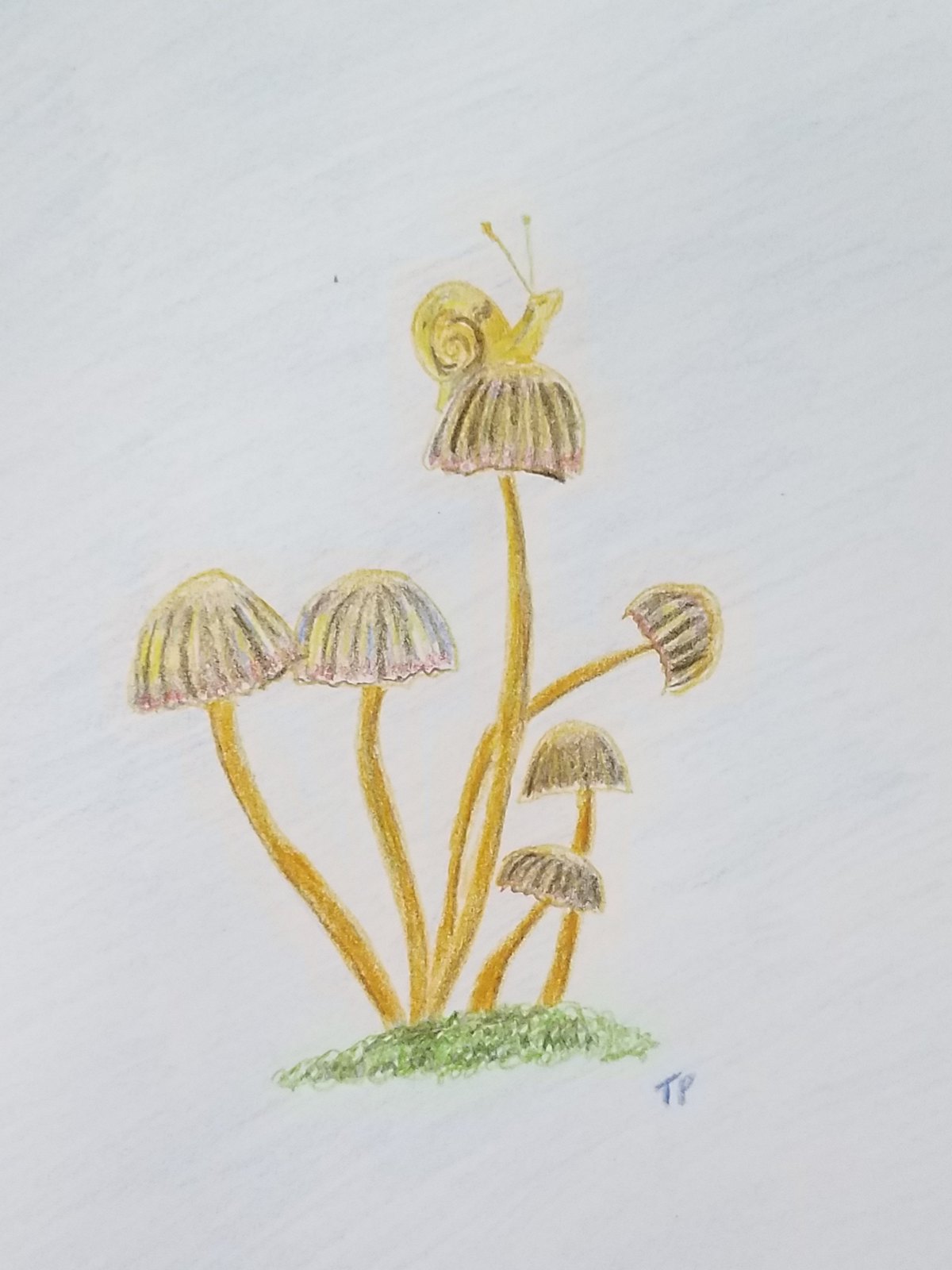The image is a detailed drawing set against a white paper background, featuring a charming scene of pastel-colored flowers and a small snail. The flowers are depicted with yellow stems, and their petals are a blend of pastel hues, primarily pink at the bottom transitioning into darker colors towards the top. Prominently perched atop the central flower is a yellow snail adorned with scattered black spots on its side. The snail's distinctive yellow antennas form a V-shape. Beneath the flowers, the grass is colored in, completing the idyllic setting. The artwork is signed with the initials "TP," likely indicating the artist.